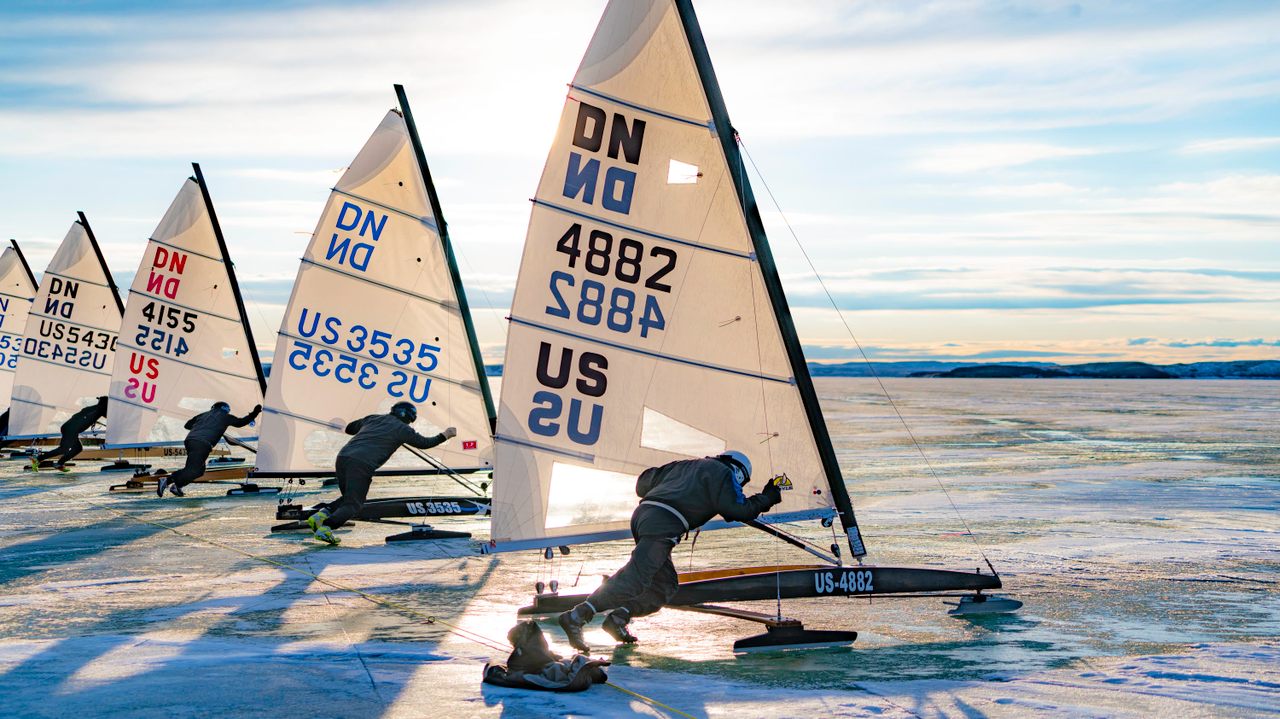The image captures the starting line of an ice sailing race on a frozen lake. The surface is covered in snow, with low hills visible in the distance under a blue sky filled with wispy white clouds. Five ice sleds, each equipped with a triangular sail, are positioned at the starting line. The sails prominently display serial numbers beginning with 'DN' followed by 'US' and unique numbers like '82' and '3535'. The sleds also feature a beam with a single ski at the front and two skis at the back, which help them glide across the ice. Sunlight shines through one of the sails, emphasizing the winter setting. The racers, all in winter gear with helmets and gloves, stand behind their respective sleds, poised to push them forward as the race is about to begin. In the foreground, possibly a dog sits on a blanket, adding a touch of warmth to the chilly scene.